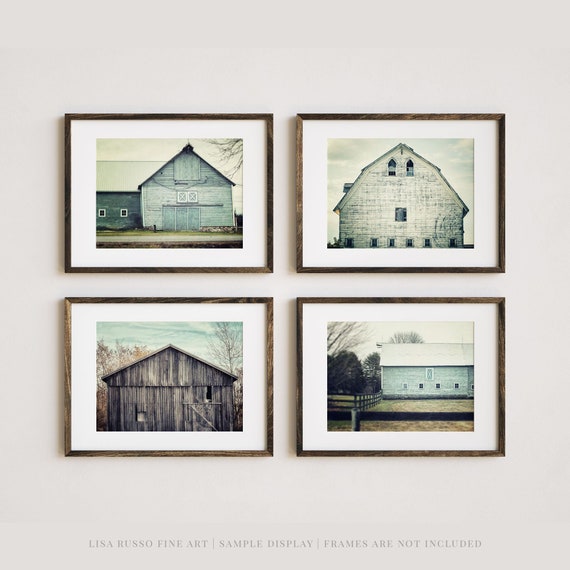The image displays four framed photographs arranged in two horizontal rows, each featuring a barn. The frames are thin black wood with white mattes around the pictures, mounted on a light gray wall. Each photograph captures a different perspective of barns, unified by their rustic, triangular rooftops.

The upper left photograph shows a gray barn with a triangular roof made of gray wood, with a rectangular section extending to the left. The upper right image presents a tall, light gray barn with a jagged, wide triangular roof and several windows. The bottom left photograph features a shorter dark gray barn with a distinctly triangular roof, set against a blue sky. The bottom right image offers a side view of a very light gray farmhouse, framed by a brown picket fence, with sky and grass or dirt visible at the top and bottom.

At the bottom of the display, text in gray reads "Lisa Russo Fine Art. Sample display. Frames are not included." The prints are evenly spaced with about six inches between them.